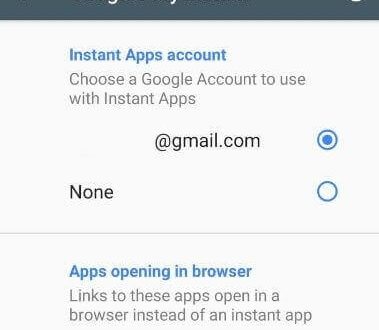The image features a close-up view of a settings screen, distinctly showcasing various elements related to the configuration of instant apps. At the top, there is a navy-blue border with white text, though the details of the text are indistinguishable due to the zoom level. 

Beneath the border, the screen transitions into a light gray backdrop, where the heading "Instant apps account" is prominently displayed in bold, blue font. Below this heading, a subtitle reads, "Choose a Google account to use with instant apps."

Under the subtitle, there is a partially redacted email address ending in "@gmail.com" with a blue filled-in dot beside it, indicating it is the selected account. Below this email address, the option "None" is listed with an unfilled blue outlined dot next to it, signifying that no other accounts are selected.

A faint gray line separates the top section from the bottom portion of the screen. This lower section is labeled "Apps opening in browser," which is written in a slightly bolder blue font. The detailed description underneath clarifies that links to selected apps will open in a web browser rather than in an instant app.